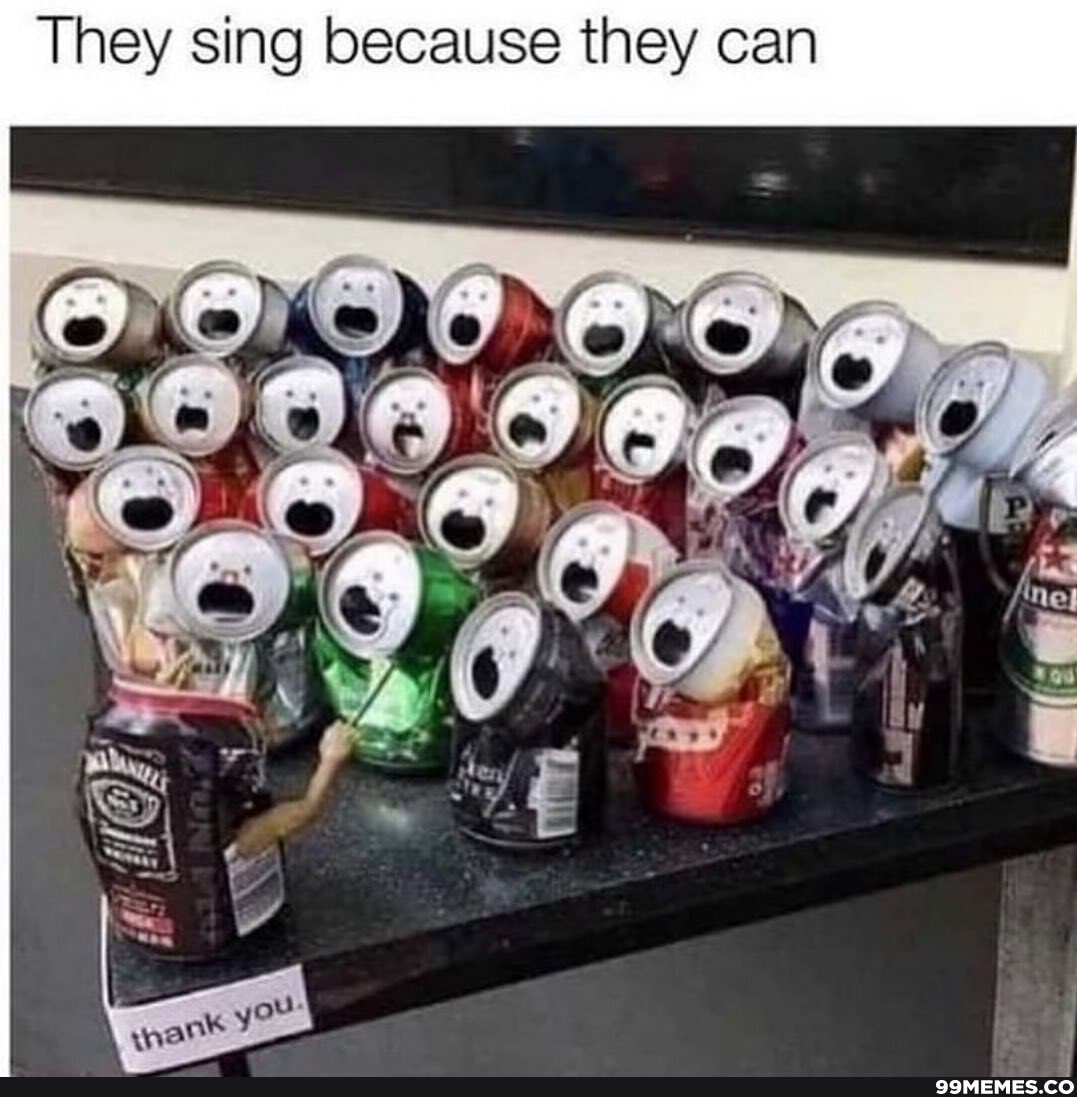This photograph depicts a whimsical scene of a choir formed entirely from empty, crushed drink cans arranged on a black table. Each can has been carefully manipulated to resemble a face, with the can's opening forming a mouth and the two tab holes appearing as eyes. The cans are positioned in rows, with the back row holding the most cans and fewer cans in each successive row leading to a trio in the front. One prominent detail is a Heineken can and a Jack Daniels can, among others colored green, red, black, yellow, and purple. In the bottom left corner, a can with a plastic toy arm, holding a conductor’s wand, appears to be conducting this makeshift choir. Above the image is the text "they sing because they can," which humorously emphasizes the visual pun. On the black table, a note of gratitude can be seen at the very corner, with the word "thank you" written on what seems to be an attached card. In the bottom right corner, the source "99memes.com" is partially visible, and the background above the table fades from white to black. Overall, the image cleverly transforms ordinary cans into a choir of singing characters, led by an enthusiastic conductor.